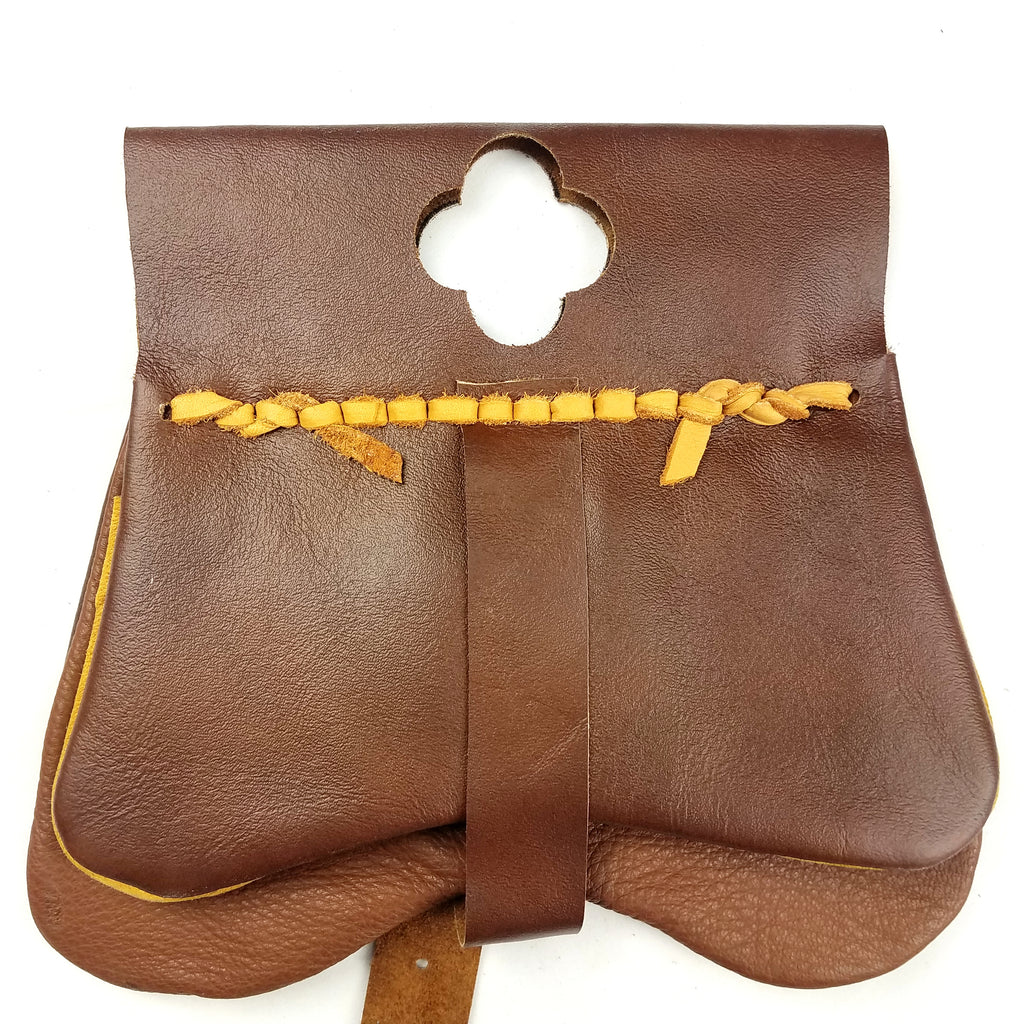This detailed photograph showcases a handcrafted leather bag set against a stark white background, emphasizing its intricate features. The bag, made from light brown leather with a smooth, shiny texture, is adorned with distinctive gold-yellow leather stitching that runs horizontally across its midsection. At the top, there's a four-leaf clover-shaped cutout that adds a unique touch to its design. A central yellow rope zigzags horizontally, while a brown leather strap vertically encircles the bag, likely serving as a clasp to secure its sides together. The bag also has a second strap, visible from behind, adding to its functional design. Despite its small and somewhat irregular shape, hinting at a handmade nature and potentially lower-quality leather, the craftsmanship is noteworthy, giving it a rustic, artisanal appeal.